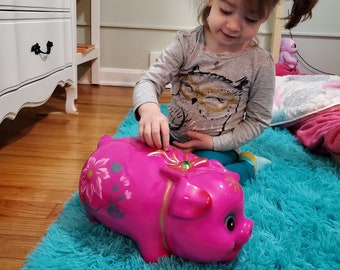This indoor photograph captures a young Caucasian girl, possibly three or four years old, as she engages with her hot pink piggy bank adorned with pink and green flowers and a gold-accented bow around its neck. The child, with her brown hair styled in a ponytail or pigtail, is dressed in a long-sleeved shirt that features a metallic screen print of an owl wearing gold glasses. Her shirt appears to be white and brown, and she pairs it with deep teal or dark gray leggings. She is seated on her knees on a bright teal shag rug, the high pile of which reflects a vibrant blue or turquoise hue. Behind her, a white dresser with visible bottom drawers and an off-white wall complete the cozy scene. The setting also includes a white blanket with some patterns, possibly a part of the girl's room decor. The moment captures her in the act of putting a coin into the piggy bank, a charming snapshot of a simple, joyful activity.